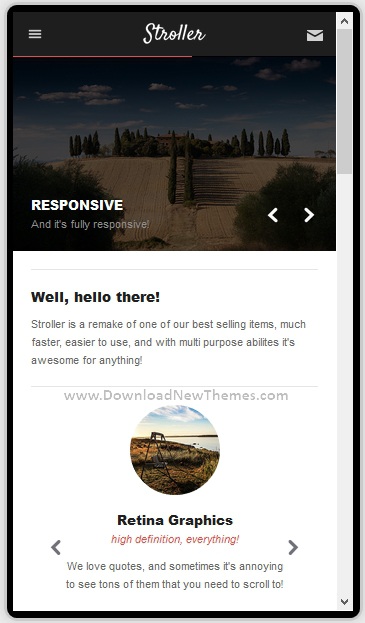This image is a screenshot captured from a mobile phone, displaying an app or website interface. At the top of the screen, the title "Scroller" is prominently featured, likely indicating the name of the app or website. Directly beneath this, the word "Responsive" is displayed, suggesting that the app or website is fully responsive to different devices. On either side of the screen, there are arrows allowing users to navigate left or right.

Below the navigation arrows, a welcoming message reads: "Well hello there. Scroller is a remake of one of our best-selling items. Much faster, easier to use, and with multi-purpose abilities. It's awesome for anything." This text highlights the enhanced features and versatility of the Scroller app or website.

Further down the screen, a URL is provided, which is www.downloadnewthemes.com, likely indicating where users can download the app or additional themes. Under the URL, a small thumbnail image is displayed, depicting a serene landscape featuring a sky, ocean view, and grassy area.

Beneath the thumbnail, a statement about the visual quality is written: "Retina graphics, high definition everything. We love quotes and sometimes it's annoying to see tons of them that you need to scroll through." This suggests the app boasts high-definition visuals and acknowledges a user experience consideration regarding excessive scrolling through content.

The entire content of this screenshot is presented within a rectangular frame on the mobile device's display.